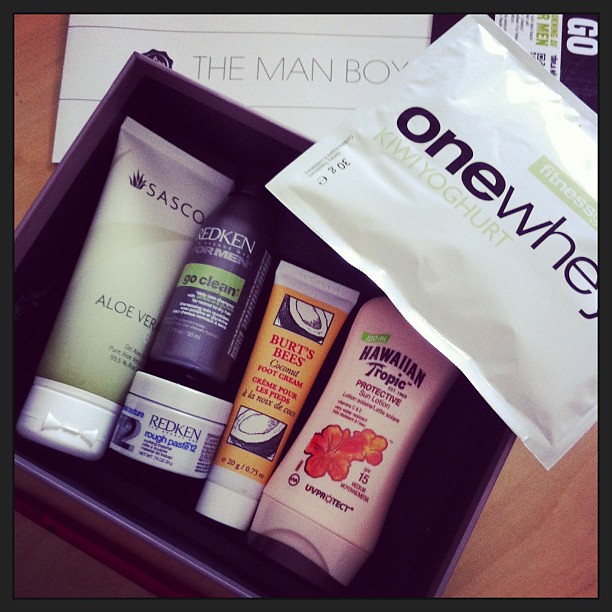The image showcases a collection of personal care products neatly arranged in a dark purple box, set atop a brown wooden surface. On the far right, there's a mostly white bottle of Hawaiian Tropic Protective Sun Lotion SPF 15, adorned with orange flowers. Beside it is a yellow and white tube of Burt's Bees Coconut Foot Cream, featuring cartoonish coconut logos. A small black container labeled Redken For Men Go Clean, in gray, black, and green hues, sits next to a round white canister of Redken Rough Paste 12. A white and green tube of Sasko Aloe Vera Gel is also visible. Above the products, there's a white package that reads "One Way Kiwi Yogurt" in a white bag or envelope. The image, likely taken for social media, appears to have a filter applied, enhancing its contrast.